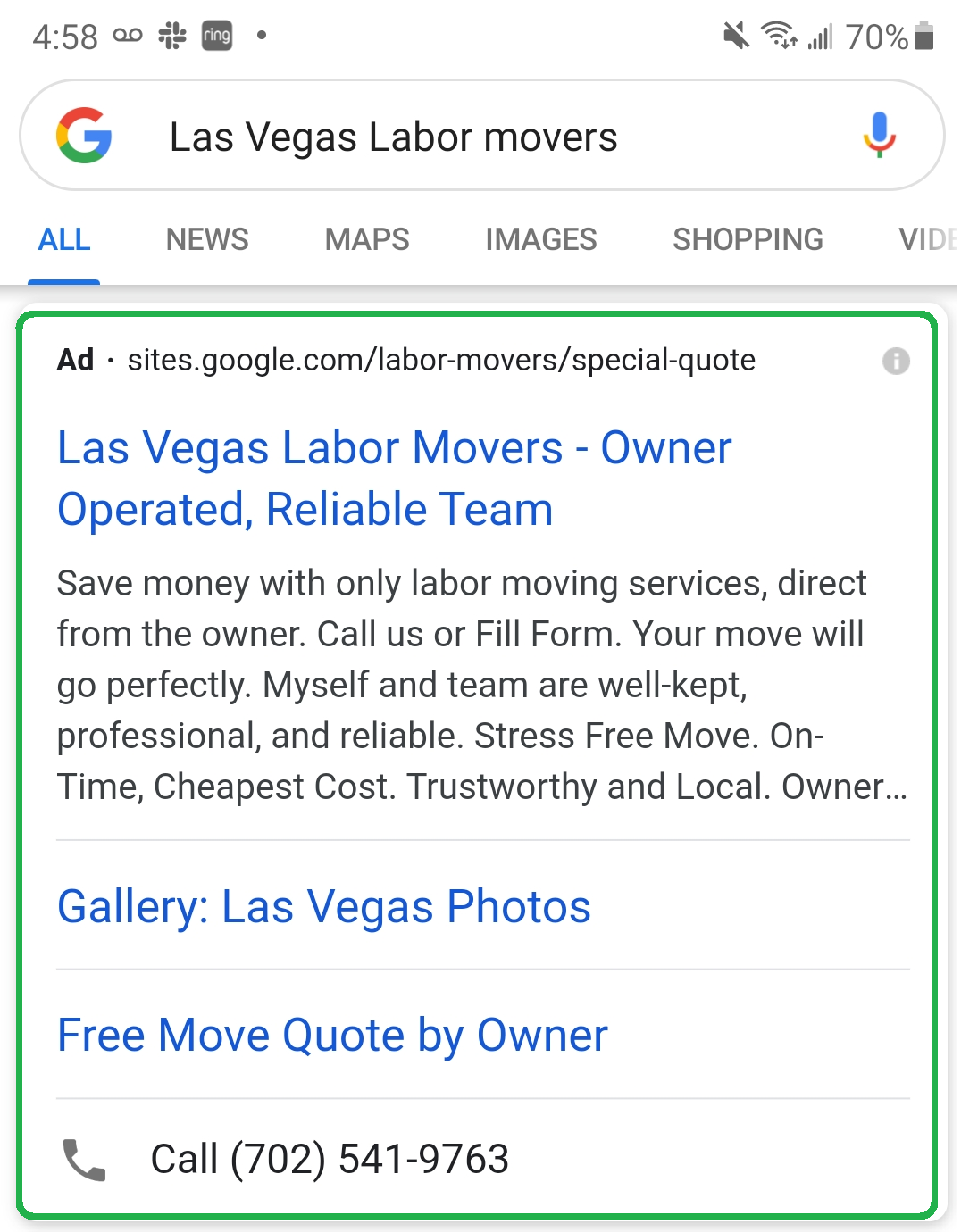A mobile phone screenshot from Google displays various icons and information at the top: a battery percentage of 70%, full Wi-Fi signal, and nearly complete mobile signal strength. Additionally, there are a variety of symbols, including an infinity sign, a flower, a square with the word "ring," and a muted sound icon. Below these icons, a Google search has been conducted for "Las Vegas labor movers." The search page shows various options like "All," "News," "Maps," "Images," "Shopping," and "Videos," with "All" selected. The top search result is an ad from sites.google.com for Las Vegas labor movers, indicating it is an owner-operated, reliable team with a tagline promoting cost-effective, labor-only moving services in black font.